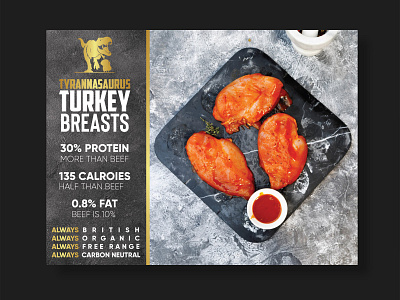In the image, there's a beautifully plated dish featuring cooked turkey breast, presented on a square-shaped black plate placed on a gray and white table. The turkey breasts appear golden-brown, doused in a reddish sauce, with an additional portion of the sauce served in a small white cup positioned at the bottom of the plate. Adjacent to the dish is an informational display. This display, framed in black, bears a vertical gray box on the left side showcasing a golden dinosaur logo and text written in golden fonts. The text reads, "Tyrannosaurus Turkey Breast" and highlights, "30% protein more than beef, 135 calories, half than beef, 0.8% fat, beef is 10%," along with the phrases, "always British, always organic, always free-range, always carbon neutral." The word "always" is particularly emphasized in a distinctive gold color. Above the text, there's a small drawing of a T-Rex running and roaring. The entire setup gives an impression of a high-quality, health-focused food product.